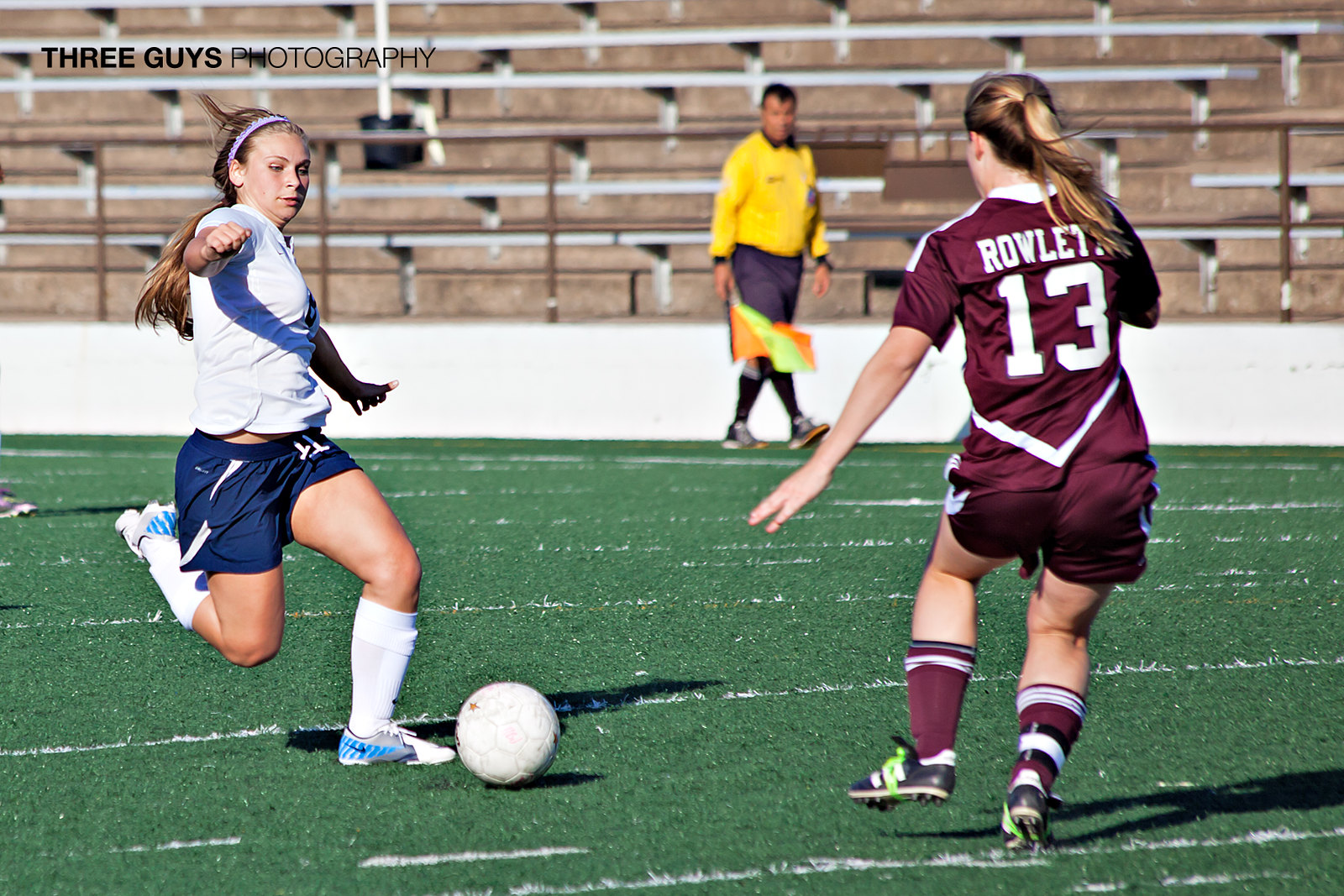In this dynamic action shot of a soccer match, two women from opposing teams are the focal point. One player, wearing a dark red jersey with the name "Rowley" or "Rowletti" and the number 13 on her back, is seen from behind. Her dark red shorts and socks with white stripes complement the jersey. Facing her, another woman is captured mid-action, her leg raised as she prepares to kick a white soccer ball. She is dressed in a white jersey, blue shorts, and white socks. The vivid green soccer field is marked by white lines, providing a sharp contrast to the players' uniforms. A sideline referee stands in the center background. He is identifiable by his bright yellow jersey and the yellow and red flag he wields, set against the backdrop of empty concrete stands. At the top left corner of the image, the black letters of "Three Guys Photography" subtly mark the frame, tying together this striking moment in the match.